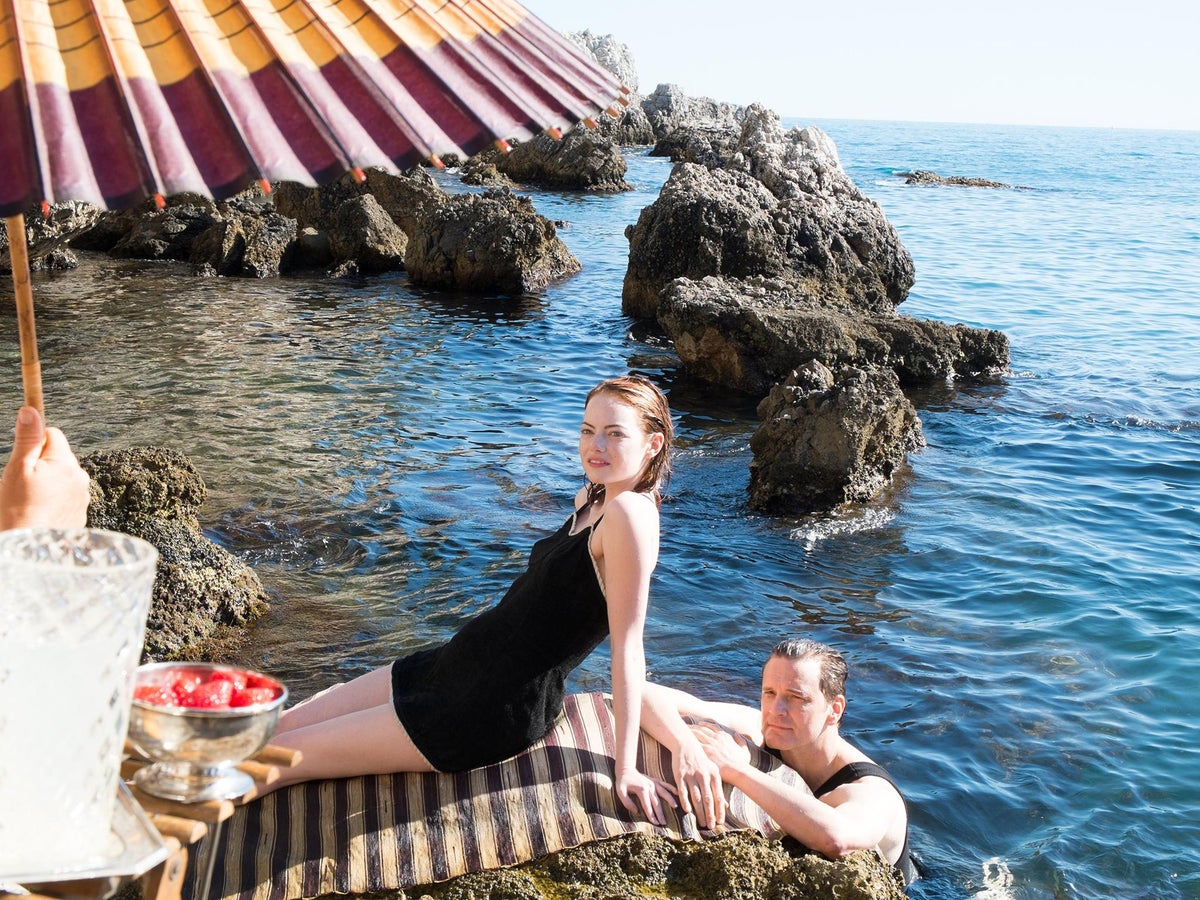In this image taken outside at a beach, you see a scene reminiscent of a movie still featuring actress Emma Stone. The sky and ocean are both a vibrant blue, while rocky formations surround the area. Emma Stone, with her brown hair cascading past her shoulders, is seated on a stone close to the water. She is wearing a black tank top and shorts, and sits on a blanket with black and beige stripes. In front of her lies a wooden table holding a plate of strawberries and a glass filled with ice. Nearby, a red and white umbrella is held by an unseen person, with only their hand visible.

In the water next to Emma, a man, possibly another actor, is submerged up to his chest. He wears a black tank top and holds onto the edge of the blanket. The calm water ensures Emma stays dry despite her proximity. The clear, daylight sky adds to the serene and picturesque setting, where the woman and man appear to be enjoying a tranquil moment at the beach.